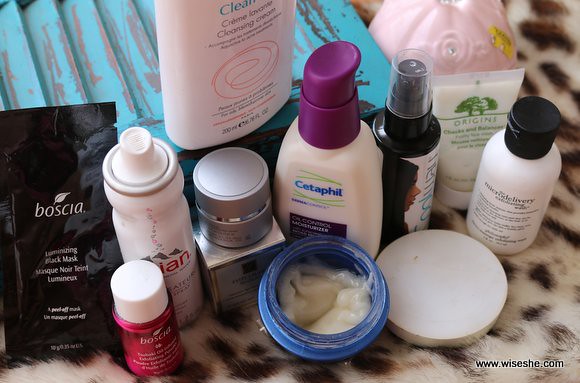The landscape-oriented image showcases an artfully arranged selection of various facial care products displayed on a plush, white leopard-print blanket adorned with brown patches. There are approximately ten different products in the frame. In the upper center, a prominent Evian spray bottle stands tall beside a small, red bottle with a white cap. In the front center, an open blue canister reveals a creamy lotion inside. Adjacent to the blue canister, a white bottle of lotion with a fuchsia cap catches the eye. To its side, a sleek black bottle with a closed cap adds contrast. Completing the ensemble, there is another lotion product packaged in a squeeze tube, and a capped lotion bottle. The array of skincare items and the luxurious texture of the fluffy blanket create an inviting and indulgent scene.